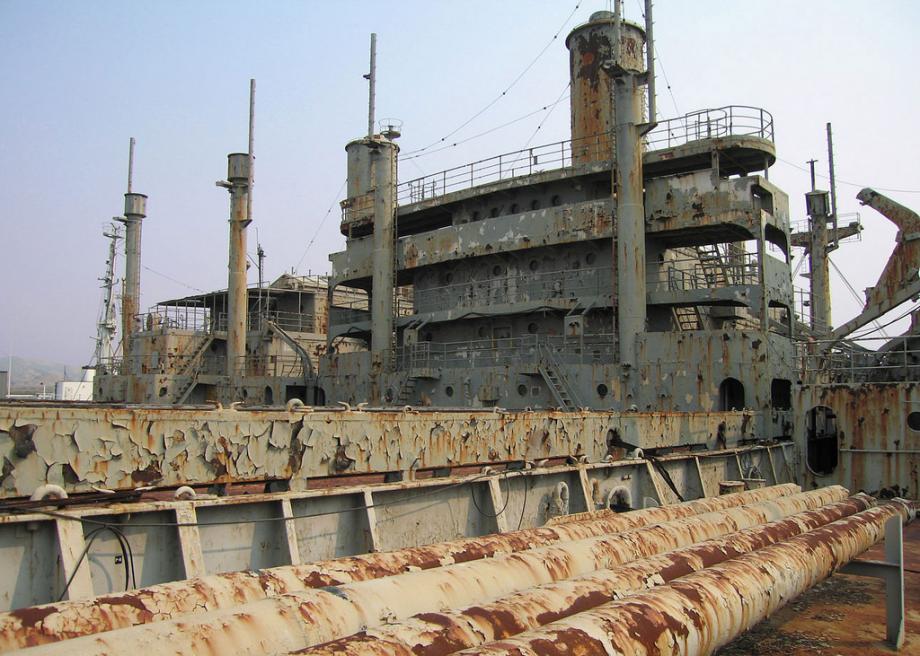The image depicts an old, abandoned facility, possibly a battleship, viewed from an aerial perspective. The entire structure is heavily rusted, with flaking metal surfaces and peeling paint in a ghostly pale yellow interspersed with pervasive brown rust. Prominently, there are at least four towers rising from the taller back section, each adorned with antenna-like structures and interconnected by wires. These towers, reaching approximately 20 feet, are situated amid the facility's four or five levels, each encircled by metal railings. Notably, there is a big central tower on the uppermost level, also rusted and featuring wires extending downwards. The decrepit structure includes a double-sided stairway on the left, leading up to the multiple levels, and also showcases rusted pipes extending from the lower left corner towards the upper right center, alongside corroded girders. The vivid blue sky and white clouds form a stark contrast to the decaying facility below, highlighting its state of extensive disrepair amidst clear natural lighting.